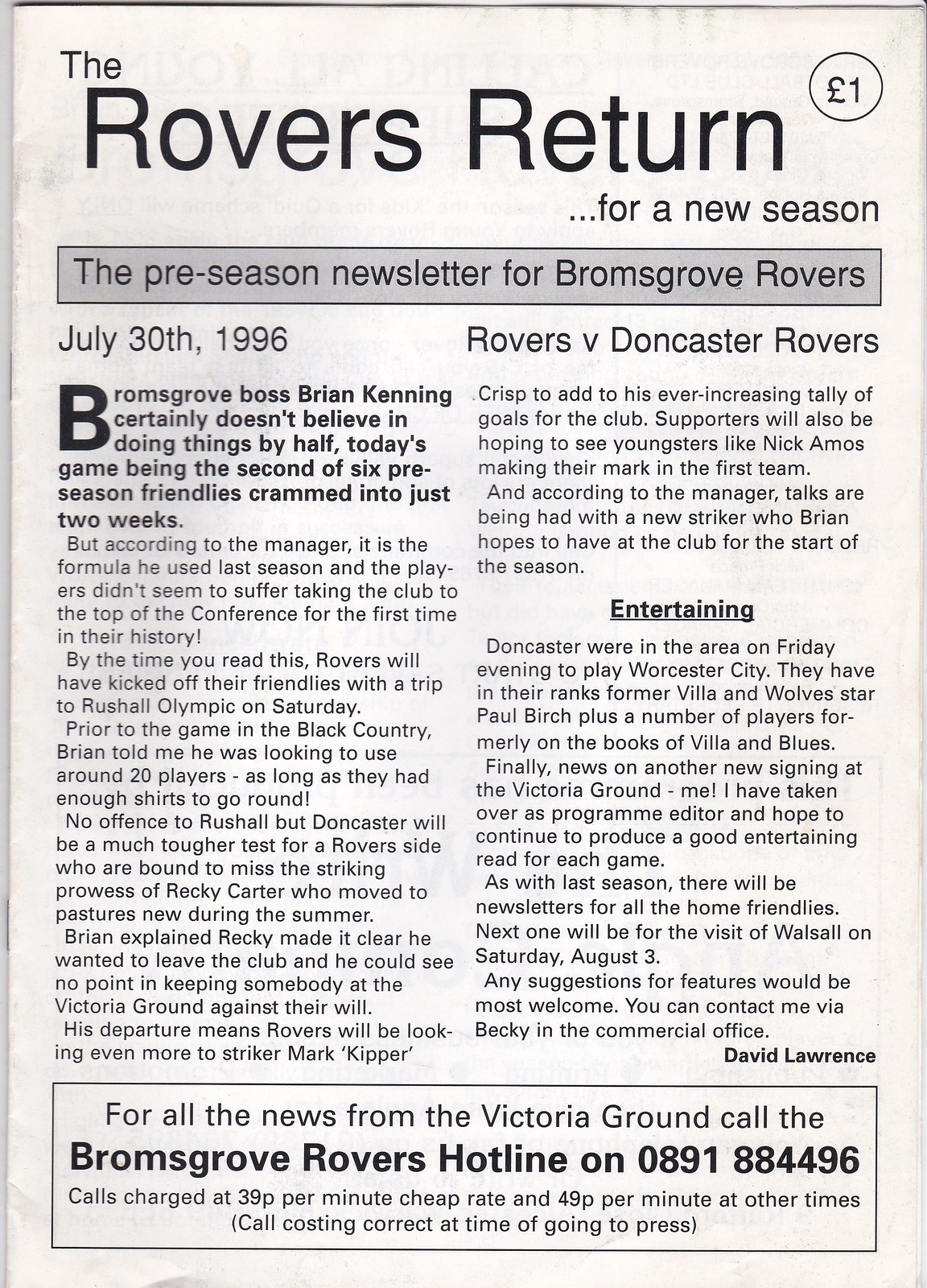The image is a black and white rectangular newsletter, prominently featuring bold black font at the top with the headline "The Rovers Return for a New Season." Below this, set against a gray bar, is the subtitle "The Preseason Newsletter for Bromsgrove Rovers," followed by the date "July 30th, 1996," and the matchup "Rovers versus Doncaster Rovers."

The first paragraph of the main article, distinguished by a darker and thicker font, reads: "Bromsgrove boss Brian Kinnings certainly doesn't believe in doing things by halves. Today's game is the second of six preseason friendlies crammed into just two weeks." The rest of the article continues in smaller print, providing further details.

Additionally, on the right-hand side of the newsletter, there is another article related to entertainment. Both articles are authored by David Lawrence.

At the bottom of the newsletter, inside a boxed-in area, it reads: "For all the news from the Victoria Ground, call the Bromsgrove Rovers hotline at 0891 884 496. Calls are charged at 39 cents per minute at cheap rate and 49 cents per minute at other times. Call costs are correct at the time of going to press." The price of the newsletter is indicated as "One Pound."

This detailed and well-structured newsletter serves as an informative preseason update for the Bromsgrove Rovers, encapsulating key details on upcoming matches and club news.